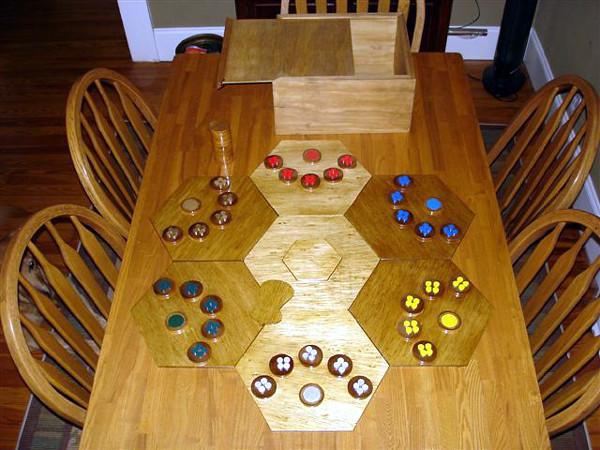This full-color photograph, captured from a top-down perspective, showcases a cozy indoor setting, most likely a living room or dining area in someone's home. Dominating the scene is a rectangular wooden table surrounded by five robust wooden chairs. The table itself sits on a wooden floor, enhancing the warm, homely ambiance of the room. 

At the head of the table is a partially open wooden box, revealing a collection of intriguing items. Spread across the table are various wooden tiles arranged in a rough pentagonal formation. Each tile is meticulously decorated with small circular discs, each flaunting a distinct pattern. These discs come in an array of colors: white, yellow, blue, red, light blue, and black. Notably, one tile in the center is devoid of any discs, offering a stark contrast to its colorful surroundings. 

Along with the tiles, there's a neat stack of additional wooden discs, suggesting the presence of a board game, likely played by those who gather around this table. The presence of these vibrant and intricately designed pieces adds a touch of whimsical charm to the scene. Additionally, off to the left side of the image, a dog can be seen, further emphasizing the warmth and lived-in nature of this home.